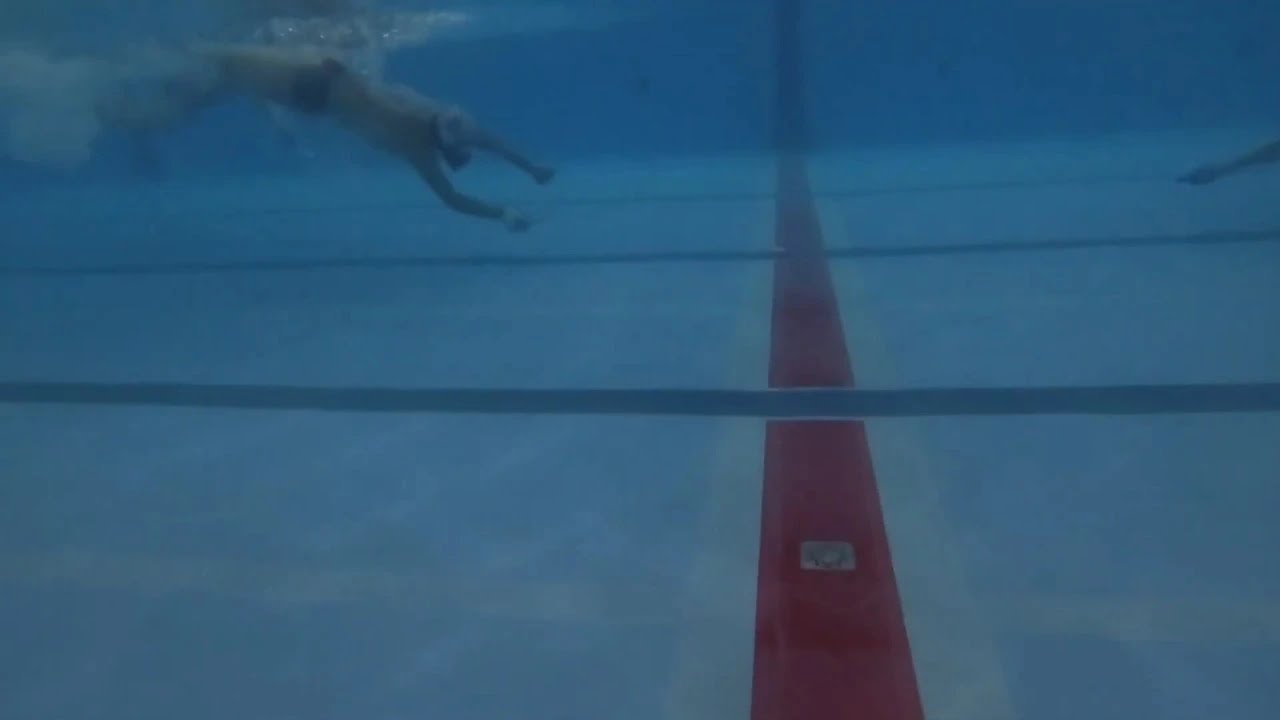This underwater image captures the dynamic setting of a swimming contest in a pool, characterized by a distinctive bluish hue typical of chlorinated water. The pool's bottom displays a variety of lines and markings: white lines positioned vertically and horizontally, demarcating lanes with darker blue stripes, and a prominent red line running through the center, extending from top to bottom with what seems like silver drainage markings. 

In the upper left corner, a swimmer is captured mid-motion, a few feet below the surface. Adorned in a small black bathing suit and goggles, he generates a flurry of bubbles and waves as he propels himself forward. His arms are angled downward, suggesting a powerful stroke. To the right of the image, an indistinct limb — possibly an arm or foot — hints at the presence of additional swimmers, likely involved in the same race but in different lanes. 

Overall, the image vividly encapsulates the excitement and movement inherent in a competitive swimming event, with its clear depiction of swimmer dynamics and pool layout.